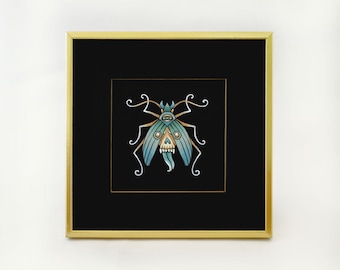This is a very small, horizontal rectangular image, depicting an intricate artwork on a lightly grayish-white background. Central to the piece is a gold frame, which encases the entire image, adding a touch of elegance. Within the frame is black matting that serves as a backdrop for the detailed focal point: a finely painted bug.

The bug, viewed from above, reveals a fascinating mix of colors and features. Its head and wings are a striking turquoise, with the wings adorned with white stripes and eye-like patterns that form the eyes of a sugar skull. The body of the bug varies, with a white central portion and distinct turquoise segments.

The legs of the insect are highly detailed, appearing gold, curly, and delicately scrolled at the ends—akin to a spider’s long, spindly limbs. This visual intricacy continues with the antennae or feelers that extend elegantly from its head, adding to its fanciful aesthetic. The bug also features pinchers and fang-like elements, enhancing its overall ornate and somewhat surreal appearance.

The overall composition, with its golden frame, black matting, and the intricate insect at the center, presents a captivating blend of natural and artistic elements, creating a visually striking piece.